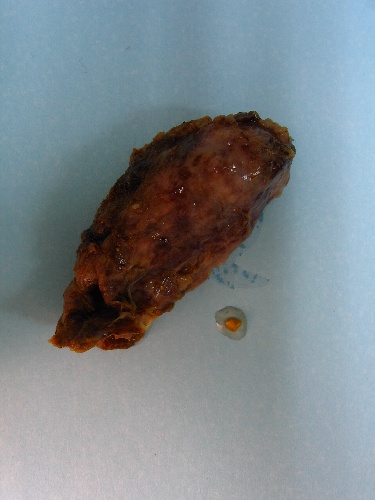The image depicts a single chicken wing, most likely fried and glazed, positioned on a white background that could be a piece of white paper. The chicken wing is a deep brownish-red hue, suggesting it is well-cooked, potentially overcooked. It is centrally located and angled slightly to the right. Underneath and around the chicken wing, there is visible grease, adding a glossy sheen to the surface. To the right of the wing lies a small piece that seems to have broken off, surrounded by a greasy spot with a tiny red dot inside, perhaps a fragment of the chicken wing. The overall color palette of the image includes the deep brown-red of the chicken wing, the stark white background, and the dark gray or blue shadows cast by the wing.